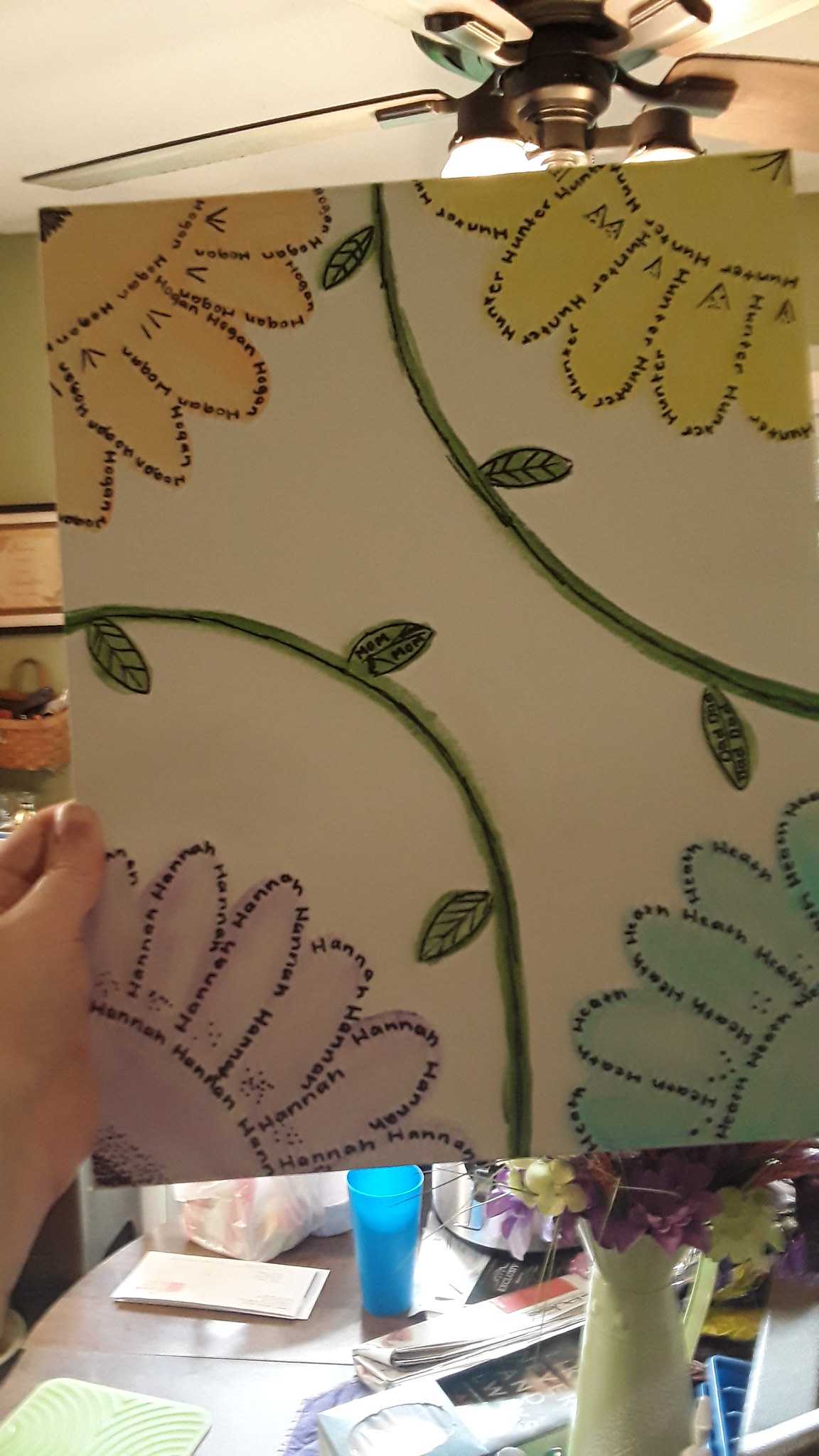In this detailed close-up photo, a diverse setting is captured. At the top of the image, there is a white ceiling adorned with a brown ceiling fan, its lights turned on, providing a warm ambiance. Below the fan, a desk is visible, appearing somewhat cluttered with various items - a blue cup, a pad of paper, a folded newspaper, and a white vase filled with flowers.

Central to the image is a left hand, presumably of an adult, holding a sturdy board. This board isn't flimsy like paper; it's firm enough to maintain its shape. Displayed on the board are four intricately detailed flowers, each occupying one of the corners.

- **Top left flower:** This flower is a very pale orange or peach color, with the name "MEGAN" (M-E-G-A-N) subtly written around its petals.
- **Top right flower:** A bright yellow flower features the name "HUNTER" (H-U-N-T-E-R) encircling its petals.
- **Lower left flower:** This flower is a light lilac shade, displaying the name "HANNAH" (H-A-N-N-A-H) around its six visible petals, accentuated by a looped stem and three delicate leaves above it.
- **Lower right flower:** A smaller flower, light blue in color, has five petals with an unreadable name inscribed around them, complemented by another stem with three leaves.

The meticulous details in the artwork and the surrounding elements provide a glimpse into a richly decorated, lived-in space.